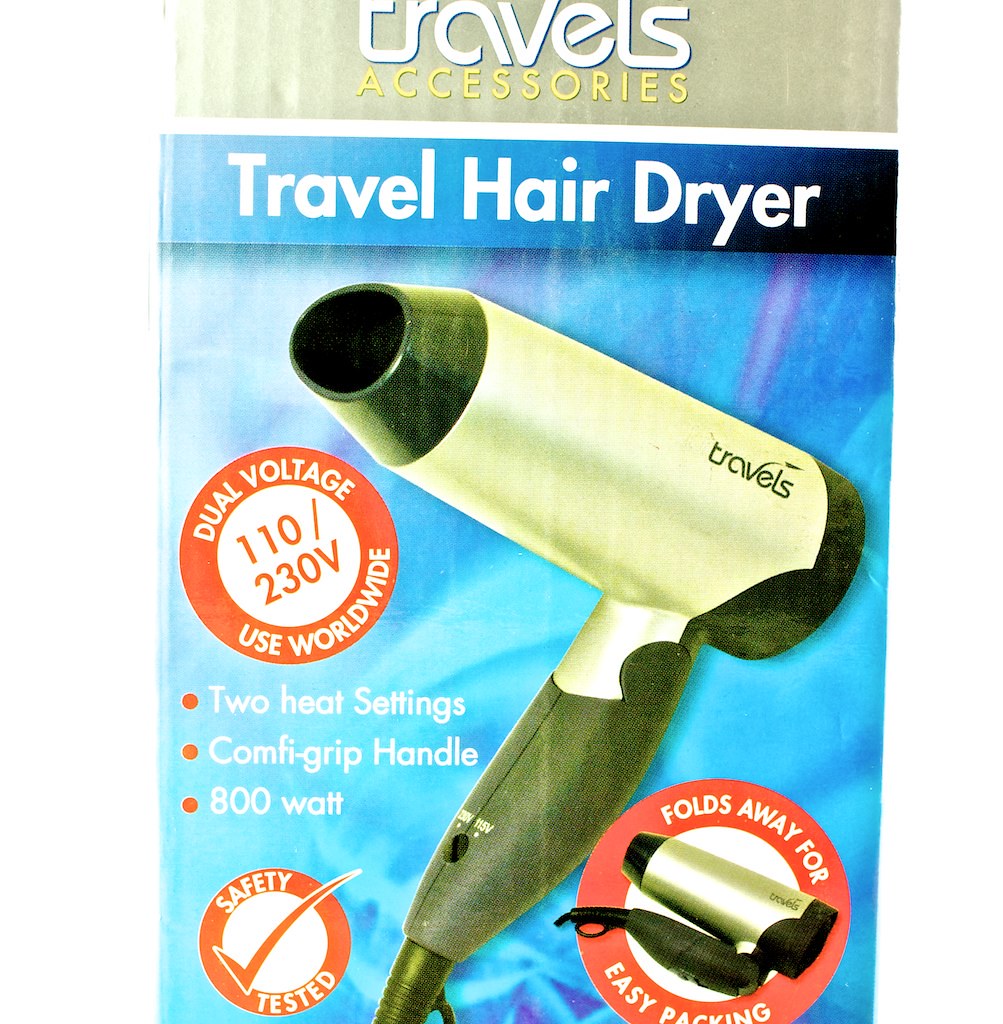The advertisement presents a travel hair dryer by Travel Accessories, showcased prominently on the front of the box. The hair dryer exhibits a sleek design with a black and silver color scheme and features attributed to its dual voltage capability (110/230V), making it suitable for worldwide use. Highlighted specifications include two heat settings, an ergonomically designed comfort grip handle, and an 800-watt power output. Additionally, the device has been safety tested, as indicated by a check mark. It is marketed for convenience with its foldable design for easy packing. The background of the advertisement displays a blue design with accents of purple and pink, although some may find the overall presentation somewhat unappealing.